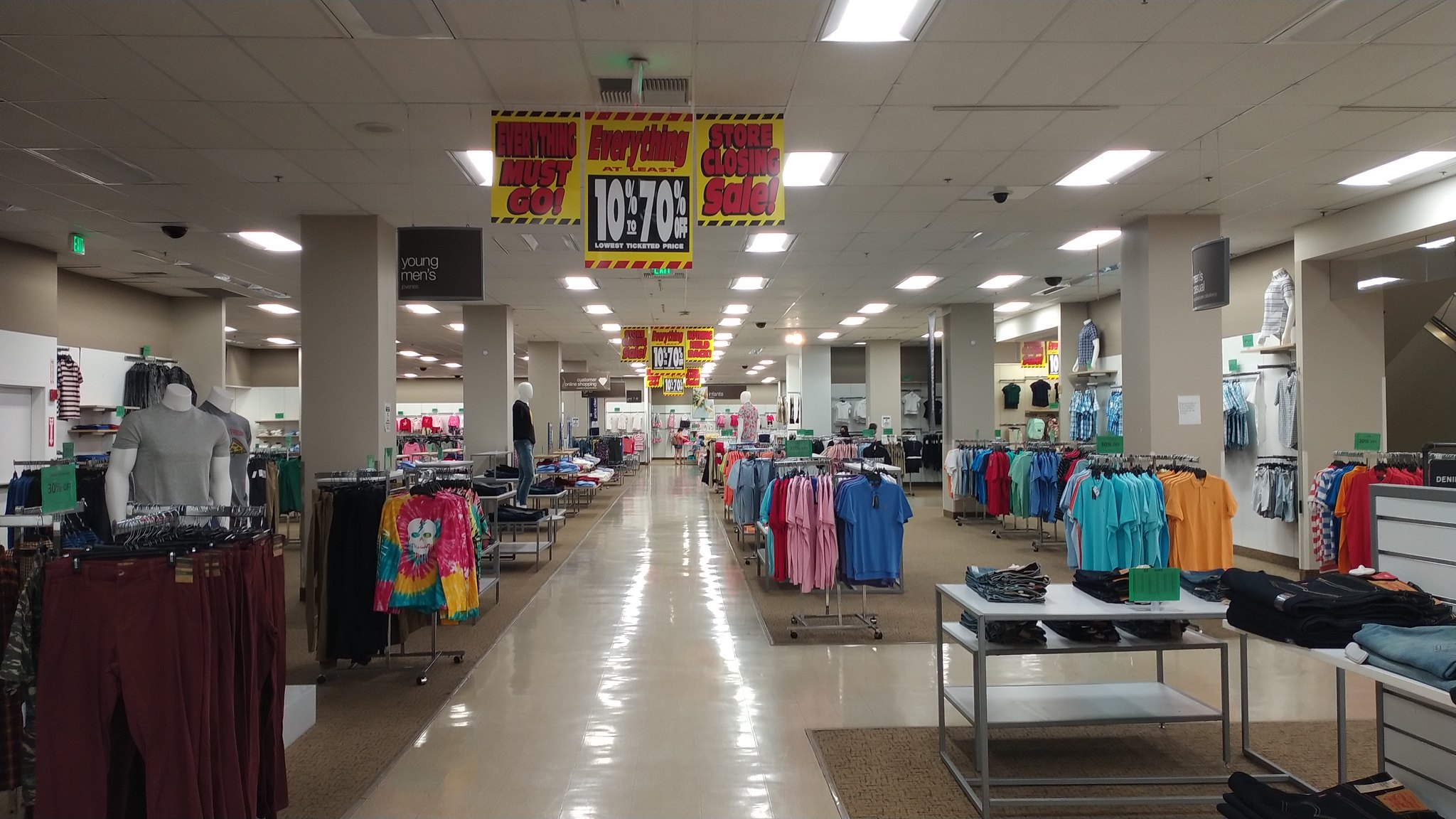This detailed color photograph captures the interior of a retail clothing store undergoing a closing sale, prominently featuring a sign hanging from the ceiling. The sign, adorned in yellow, red, black, and white, announces "Everything Must Go! 10% to 70% Off," highlighting the store's significant discounts. The store's tan linoleum floor reflects the bright overhead lighting, adding to the organized and spacious feel of the environment. 

A variety of apparel is meticulously displayed across the store, with rows of clothes that include plain gray shirts on mannequins, a tie-dye shirt featuring a skull, brown pants, and an assortment of colorful t-shirts in hues such as pink, blue, light blue, orange, and striped patterns. The right-hand side of the store reveals a fitting room for customers to try on their selections. The layout is further divided by pillars that segment different sections, and there are white shelves holding blue and black denim jeans. This organized display underscores the urgency of the sale with the bold, eye-catching signage reminding customers of the unbeatable discounts due to the store's imminent closure.